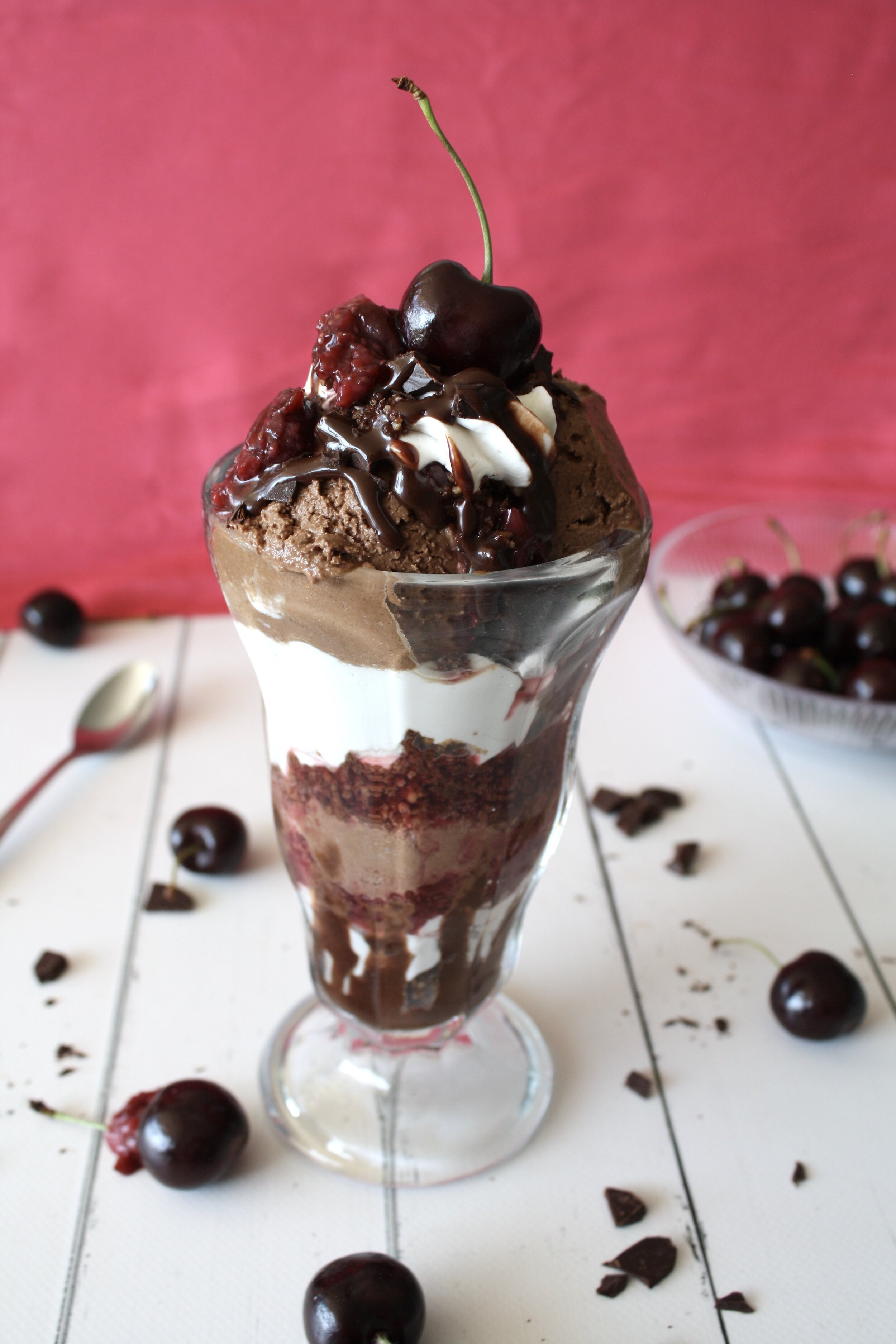The photograph captures a sumptuous chocolate and vanilla ice cream sundae presented in a classic tall sundae glass. The dessert showcases multiple layers starting with a base of rich chocolate ice cream followed by a layer of creamy vanilla ice cream, all interspersed with decadent chocolate syrup and sprinkles. The sundae is crowned with another luscious layer of chocolate ice cream topped with a glossy cherry complete with its green stem, drizzled with chocolate syrup and perhaps adorned with nuts or dried fruits. The glass is situated on a flat, white table made of long painted panels with gray grouting in between. Surrounding the sundae, the table is decorated with scattered fresh black cherries and a glass bowl filled with more cherries is placed on the right side. A silver spoon lies slightly out of focus in the background to the left. The entire scene is well-lit and set against a vivid red backdrop wall, creating a striking contrast that highlights the vibrant colors of the dessert and cherries. The parfait is generously filled, looking untouched and ready to be savored.